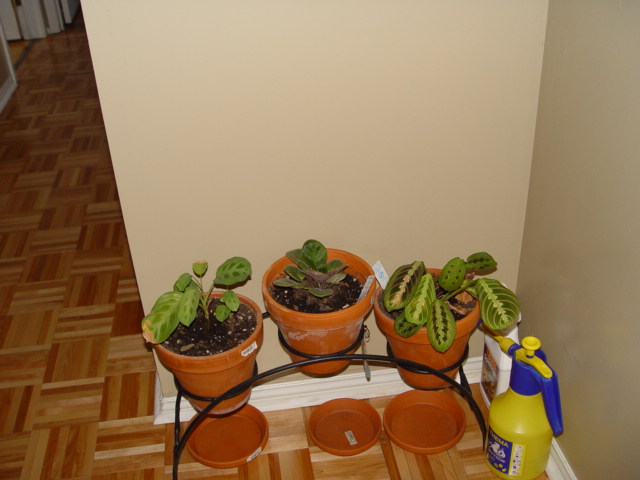This photograph captures a cozy corner of an open-plan room showcasing a charming arrangement of three potted plants. The corner features a beige wall adorned with a white skirting board. The flooring is a striking parquet pattern with wooden tiles laid in alternating directions, adding a dynamic touch to the space. The plant stand is designed in a semicircular shape, holding three terracotta pots of equal size, each equipped with a saucer underneath to catch excess water.

The potted plants display a variety of green foliage, with one plant exhibiting intriguingly patterned leaves tinged with purple. The other two plants appear to be newer, revealing more of the soil in their pots. Positioned to the right of the plant stand is a yellow spray bottle with a blue top and nozzle, likely used for watering or fertilizing the plants. This inviting indoor garden nook is a testament to the homeowner's care and attention to their green companions.